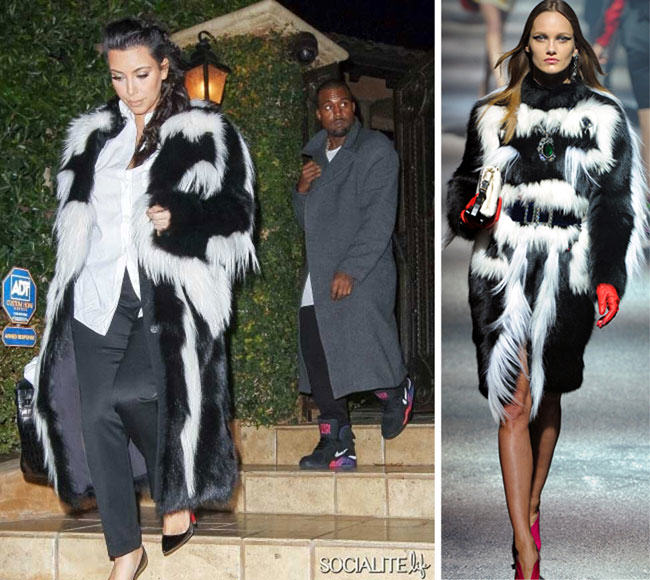In this detailed montage from Social Life Magazine, a captivating scene unfolds at night, featuring an outdoor setting with Kanye West and Kim Kardashian, possibly exiting a home adorned with ADT signage amidst shrubbery, or perhaps leaving a restaurant. Kanye is dressed in a gray long jacket, black pants, Nike shoes, and a white T-shirt, exuding a casual yet chic vibe. Kim, meanwhile, mirrors fashion from the runway by donning a striking black and white fur coat, reminiscent of skunk patterns, over a white shirt, black pants, black heels, and accessorized with a black purse. An additional image showcases a model wearing the same fur coat on the runway, accompanied by red heels, red gloves, and a white purse, which emphasizes the coat's fashion parade origins. The scene is candidly lit by a nearby street lamp, capturing the duo descending tan stone steps, with a backdrop of a lush, green wall. Interestingly, a man gazes off-camera, further adding to the paparazzi charm of the photographs. The images are untouched with no text, allowing the visual narrative and fashion statements to stand out prominently.